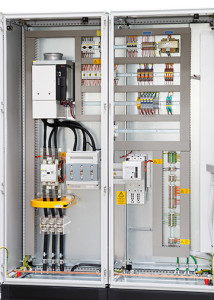The image portrays the interior of an industrial electrical compartment, with a horizontally aligned rectangular frame. Inside the compartment, there are two adjacent vertical rectangular sections. On the left side, a larger white box is positioned at the top, with black wires trailing down vertically into a series of switches beneath it, extending all the way to the bottom of the section. The right side features a complex arrangement of components, including four horizontal rectangular sections at the top, each containing different types of switches and circuits. Additionally, there is a vertical compartment on the right that also contains circuits and switches. The entire setup is encased in what looks like a white metal cabinet. The compartment is viewed through two panes of glass bordered by a silver frame, although it's unclear if these are windows or doors. This detailed structure suggests an intricate and organized electronic system, typical of industrial equipment or fuse boxes.